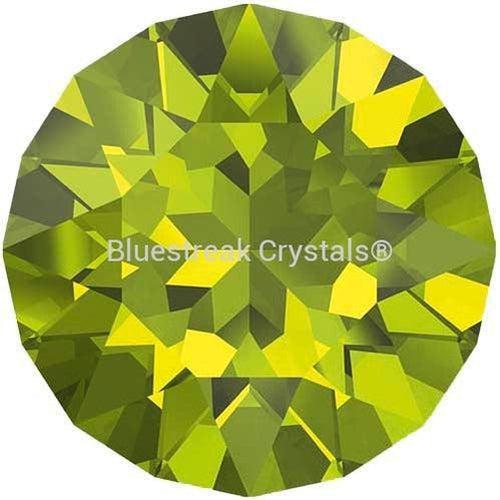The image features a computer-generated, circular gem that resembles a crystal viewed from above, with notable text in the center reading "Blue Streak Crystals," accompanied by a registered trademark symbol. The gem has a yellowish-green hue, reminiscent of the color of peas, with hints of yellow, white, and black, creating a range of reflective hues. The crystal is faceted with multiple shapes, including triangles, squares, pentagons, and hexagons, giving it a complex, intricate design. The facets project in various directions, mimicking the way light reflects off a real gem. Despite its translucency, the crystal is not very transparent and appears large, though no reference scale is provided for size comparison.